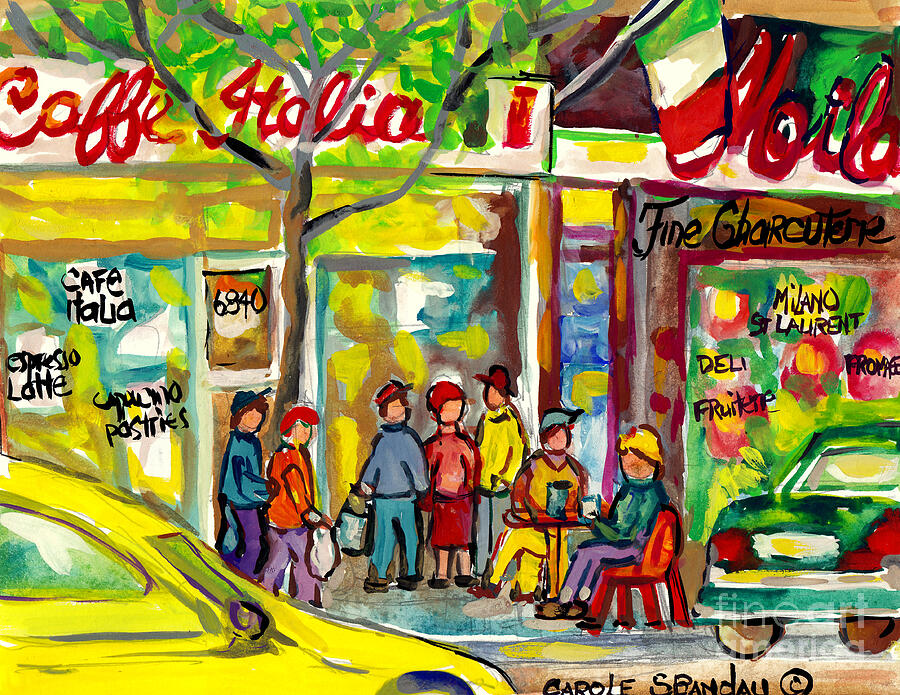This vibrant and colorful painting by Carol Spandau depicts a lively Italian neighborhood street scene. The artwork, childlike yet skillfully done, showcases storefronts brimming with activity. Dominating the scene is a thin tree with green leaves, positioned centrally. To its left, the red cursive sign "Cafe Italia" stands out on a building with an address number "6840" above the door, advertising "Espresso Latte, Cappuccino, Pastries." In front of it, five people are standing, and two are seated at a small table, enjoying their drinks. To the right, the adjacent storefront, "Muella Fine Charcuterie" with partial signage — including "MOIL" and "find" — adds more character to the scene. Cars painted in yellow and green are parked along the street. The left corner of the painting is slightly cut off, revealing most of the artist's name, "Carol Spandau," accompanied by a copyright symbol. The entire scene captures the essence of a bustling, colorful street filled with the vibrancy of daily life and the warmth of an Italian café.